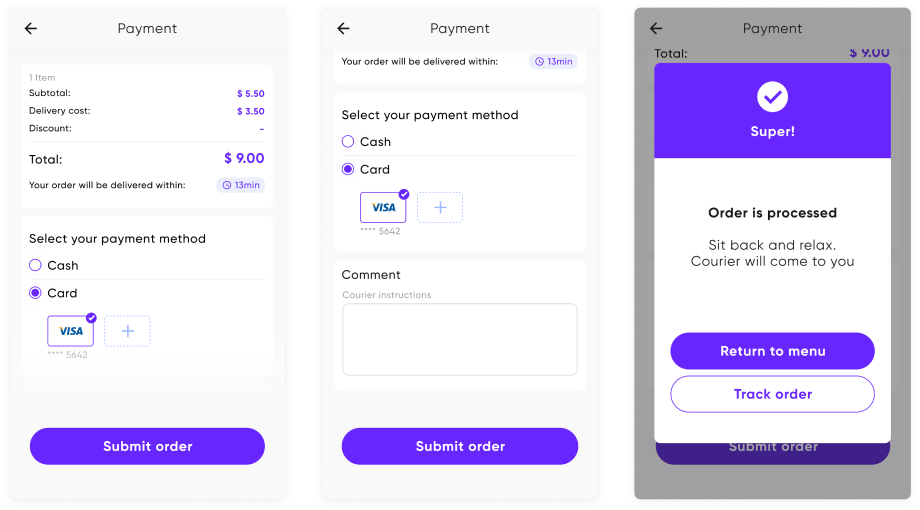Screenshot 1:
A detailed view of a payment window shows up on the left side of the screen, with "Payment" prominently centered at the top. The window is divided into two distinct sections. The first section contains a breakdown of charges in a box that lists the subtotal ($5.50), delivery cost ($3.50), a discount (not noted), and a total of $9. Below the total, a message indicates that the order will be delivered within 13 minutes. The second section is dedicated to payment options, displaying choices between "Cash" and "Card," with the card option selected, highlighted by a purple bubble. A Visa logo is shown here, along with a partially obscured card number (XXXX-XXXX-XXXX-5642) and a purple checkmark in the top right corner signifying selection.

Screenshot 2:
This image is similar to the first but includes an additional comment section just below the payment details. Here, users can input special instructions for their order. At the bottom of this input box lies a prominent purple "Submit Order" button.

Screenshot 3:
In the third screenshot, the familiar payment window is overlaid by a pop-up message, dimming the background to emphasize the prompt. This foreground message features a purple header with a checkmark and the word "Super." Below the header, the window transitions to white and boldly states "Order is processed." Additional text encourages the user to "sit back and relax, courier will come to you." The window presents two action buttons at the bottom: a purple "Return to Menu" button and a white "Track Order" button, the latter highlighted by its purple text and outline.